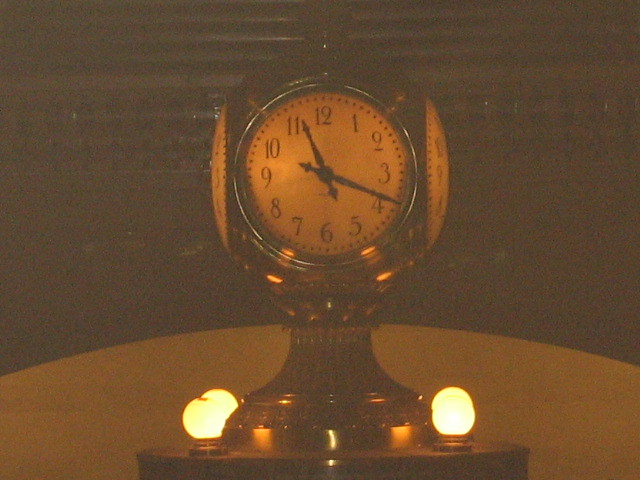This photograph features a unique spherical clock with multiple clock faces, each visible on different sides of the sphere. The clock is mounted on a circular metal pedestal with a bronze or copper-like finish, elevating it above a flat platform. Four glowing yellow light bulbs, arrayed symmetrically around the base, illuminate the scene. The clock faces display black numerals from 1 to 12 and black hands, currently indicating the time as 11:19. The faces appear in a yellowish to orange-ish hue, though this may be due to the photograph's color tones rather than the actual color of the clock. The background of the image is a dark gray to black gradient, focusing attention on the clock's intricate design and elegant form.